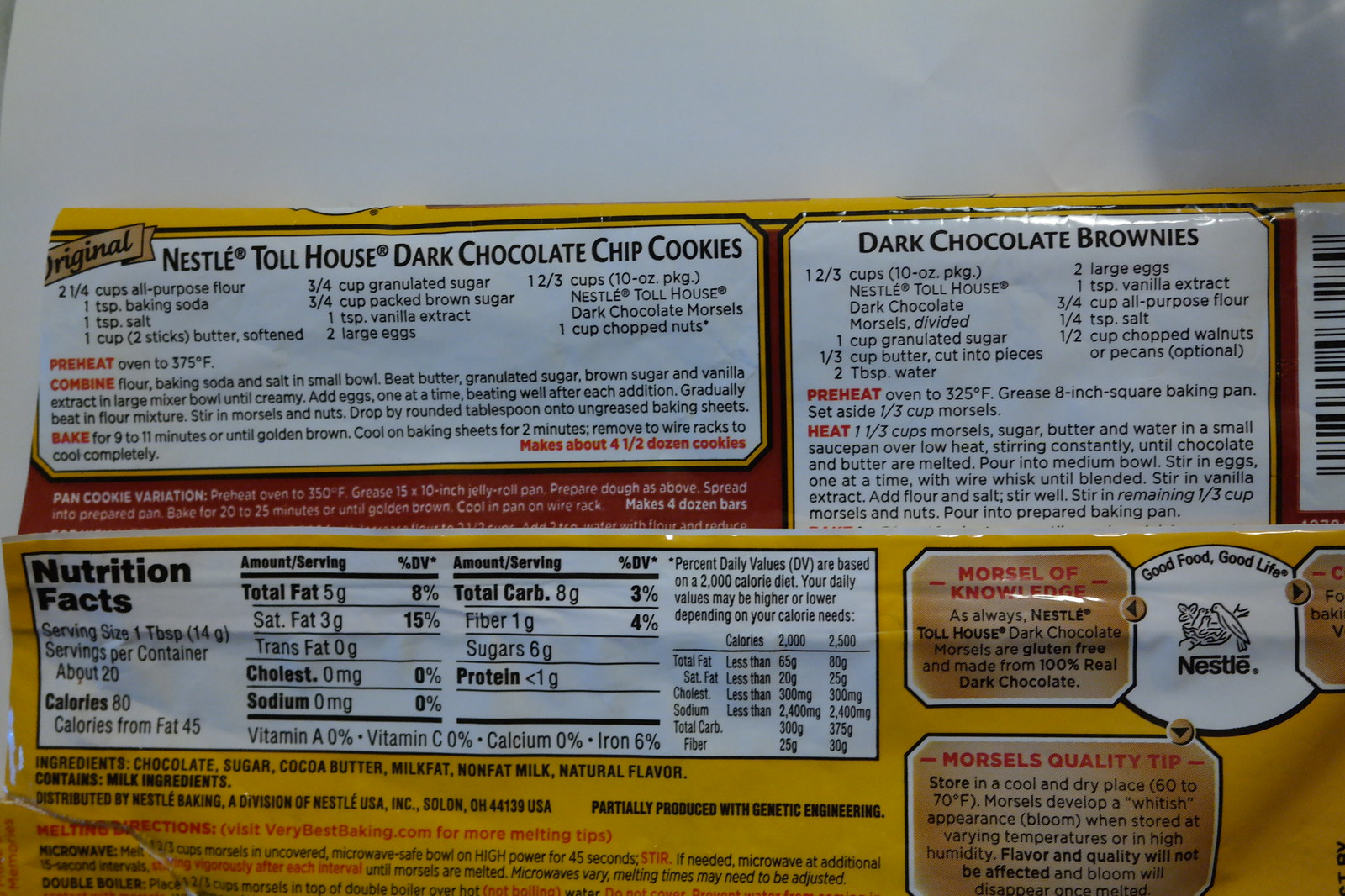This image shows the back of a Nestlé Toll House dark chocolate chip cookies packaging. In the top right corner, there's a cut-off UPC barcode running vertically. Below the UPC, there's an emblem indicating that the product contains ingredients partially processed with genetic engineering. 

On the top right section of the label, there’s a recipe for dark chocolate brownies. To the left of this recipe, you can see the white Nestlé logo accompanied by the phrase "Morsel of Knowledge." This section contains information about the brand's background. Beneath this, there’s a quality tip on how to store the chocolate morsels.

Occupying the central portion is an ingredient list and nutrition facts for the product, typical for food packaging. This detailed layout gives a clear overview of Nestlé’s commitment to providing both culinary inspiration and essential product information.